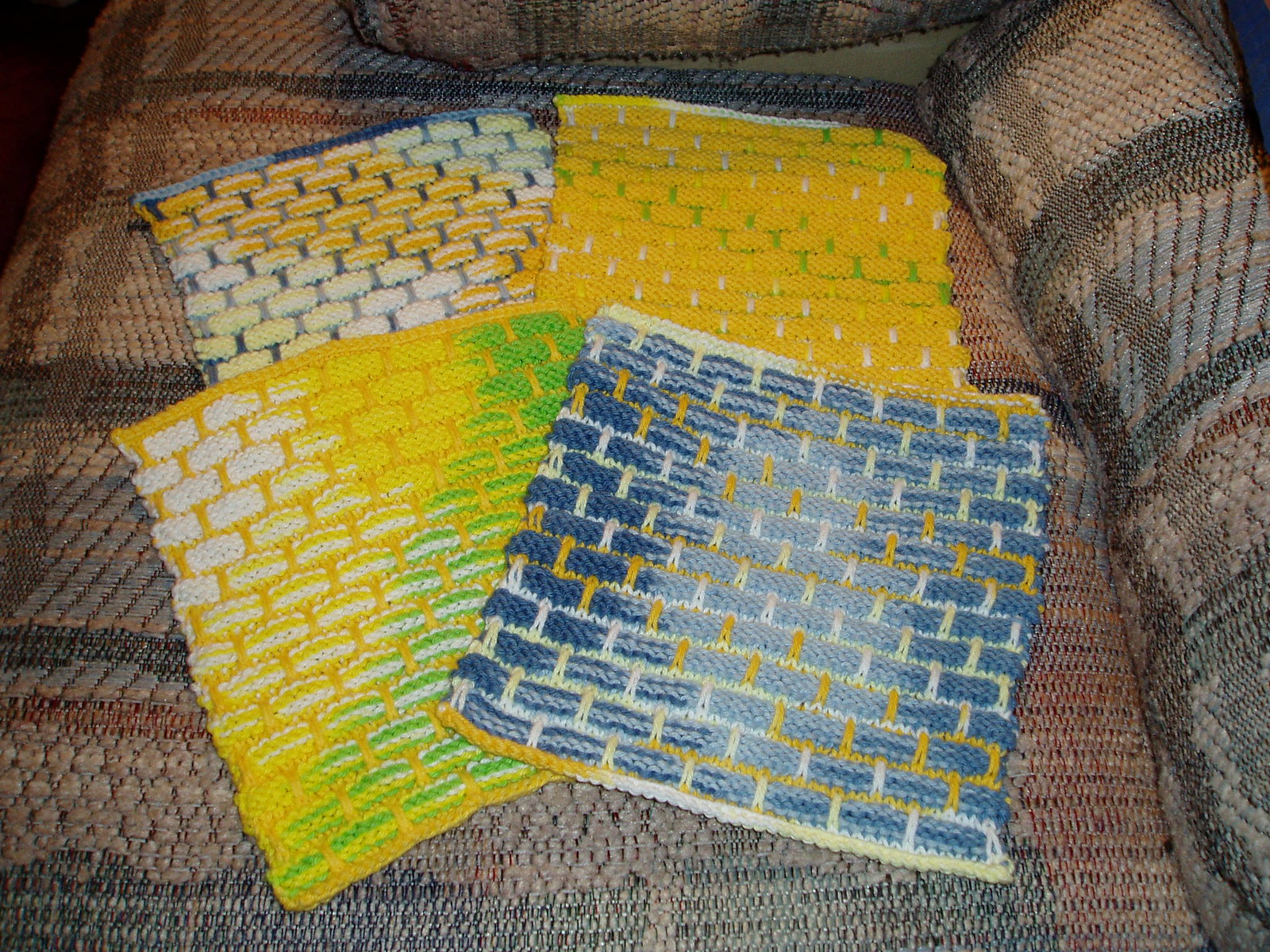This is a color photograph showcasing the base seating area of a dark brown woven couch. The upholstery features a pattern of light creamy squares with gray and blue lines. In the central part of the image, there are four vividly crocheted squares, each unique in their transitioning colors and shades, suggesting they might be potholders, placemats, or pillow covers. They are laid out in a precise arrangement: the top left square is predominantly white and yellow, while the square to its right is primarily yellow. Beneath this yellow square is another one with a blue, white, and yellow color scheme. The bottom left square features a mix of red, white, and green with hints of mustard yellow along its edge. These squares display a brick-like pattern, with varied internal colors including blues, whites, yellows, and greens, and contrasting outlines in yellow and white. In the background, parts of the couch's armrest and back are visible, framing the colorful array.